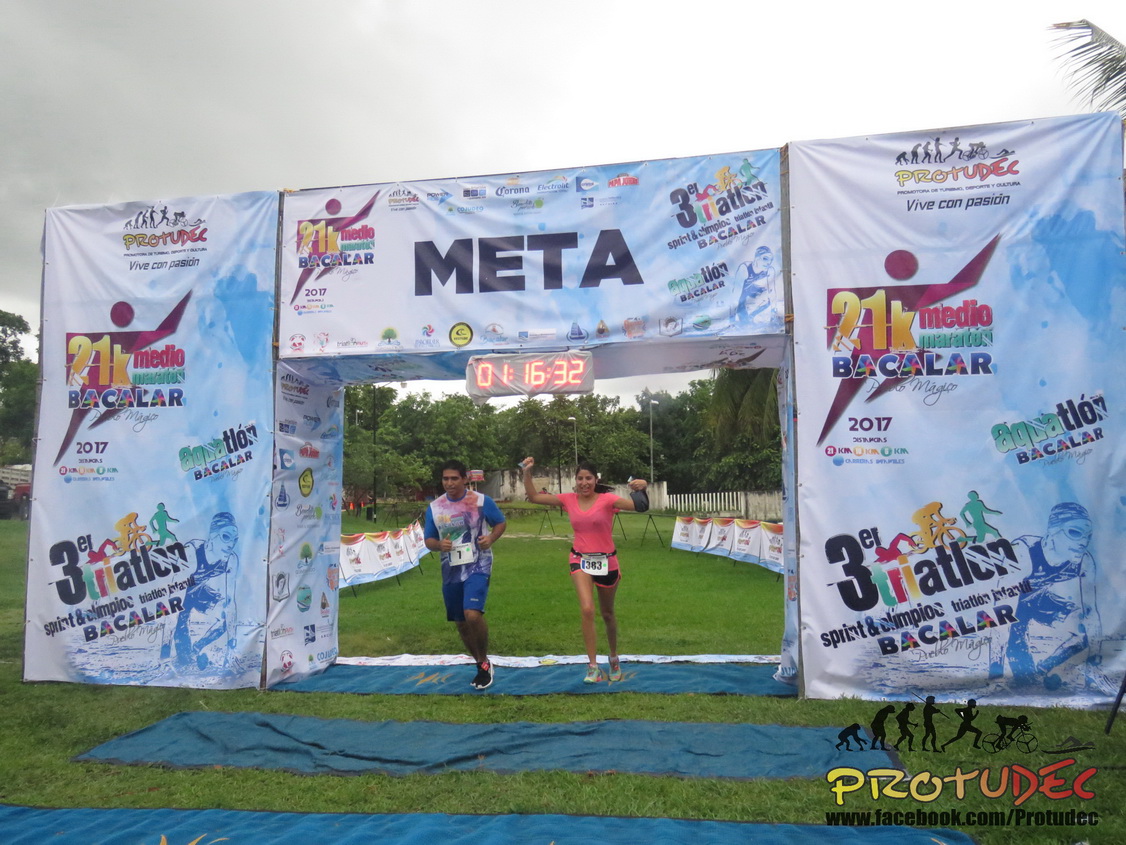The photograph captures the exhilarating moment at the finish line of what appears to be a triathlon or marathon event, marked by a prominent white cloth draped over an iron structure. This structure, adorned with colorful sponsorship logos and the word "META" in bold black letters at the center, signifies the end of the race. Positioned beneath a clock displaying the time 01:16:32 with bright orange numbers, a man and a woman are seen triumphantly crossing the finish line. The woman, clad in a pink shirt and black shorts, raises her arms in victory, while the man beside her, focused and determined, wears blue shorts paired with a blue and white top. Both runners prominently feature bib numbers. Surrounding them is a lush grassy area dotted with green trees, suggesting a vibrant, sunny day. The event banner also features text indicating "Baccalauréat 2017" and "21K Medio," hinting at a possible Spanish or Portuguese locale and suggesting the endurance of the athletes in this challenging race.